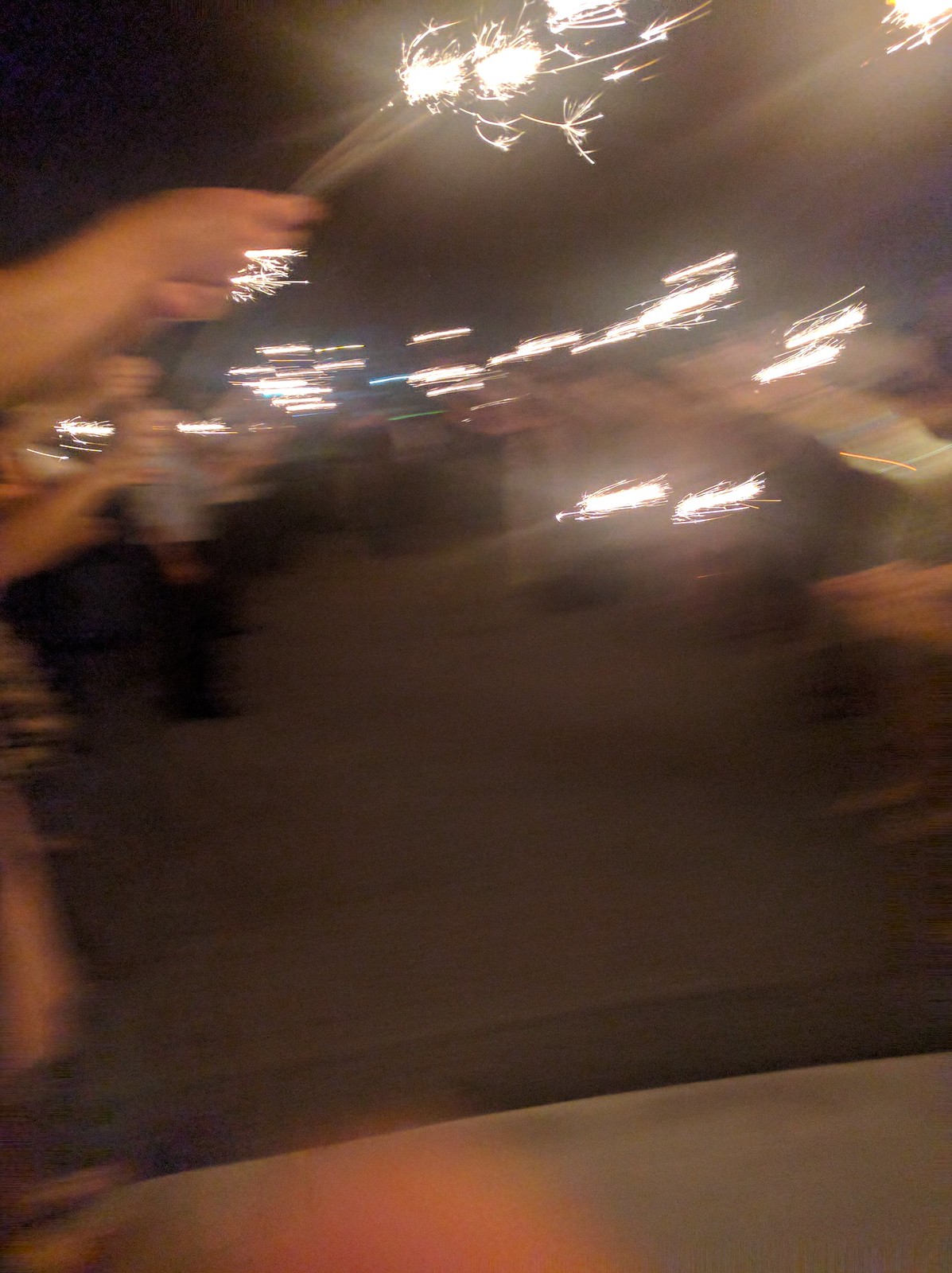The photo depicts a nighttime scene at an outdoor party with a large group of people holding sparklers. The image is very blurred, likely due to camera movement during the capture, creating an artsy, time-lapse effect. People line both sides of the frame, their hands raised and waving sparklers that appear as sparkling trails of light, resembling snowflakes. Despite the overall blur, a few details stand out: hands holding multiple lit sparklers, swinging them through the air, contributing to the dazzling yet unclear visual. The dark background and minimal colors enhance the prominence of the vibrant sparkles, emphasizing the lively and festive atmosphere.